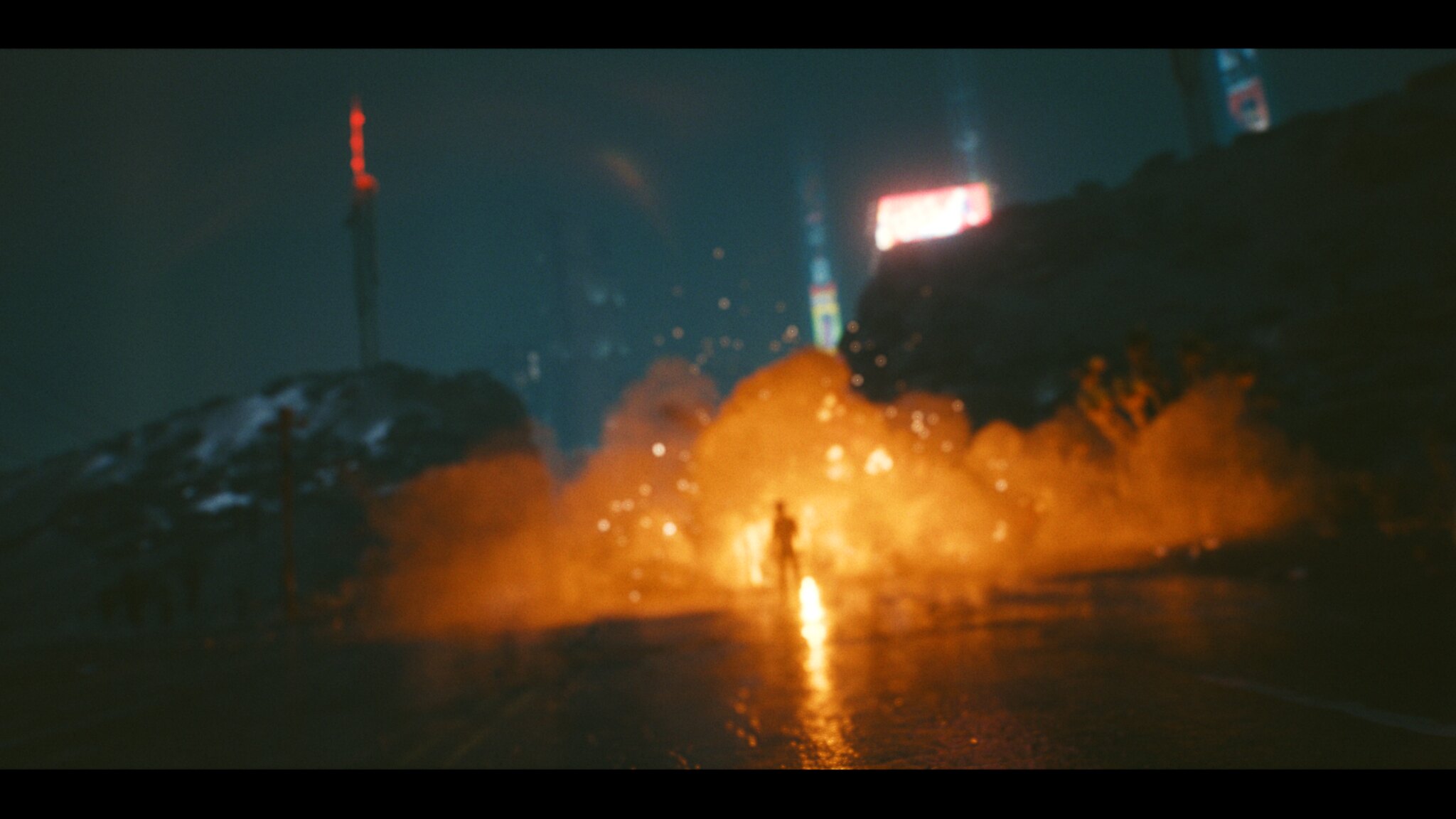The image depicts a dramatic nighttime scene reminiscent of a movie or a video game with a widescreen format, evidenced by the black bars at the top and bottom. The setting appears to be a remote area near mountains or hills, shrouded in darkness. Central to the image is a massive explosion, characterized by a reddish-orange fireball with white sparks and debris flying everywhere, illuminating the surroundings. Standing stoically in front of the explosion is a silhouette of a person, identifiable as a man by his distinct shape, yet lacking visible facial features or hair details.

On the left, there are vague outlines of trees and power lines or poles, possibly with an antenna atop a hill, while the right side features a similarly obscure hill or mountain. In the background, the landscape includes faintly lit structures that could be buildings or telephone towers, with one particularly distant structure brightly lit, possibly with a screen or advertisement, casting a neon pink hue. The sky above the fiery scene fluctuates between dark gray and faint white patches, shrouding the area in a mixture of smoke and natural night colors. The overall atmosphere suggests a backwoods road or a mountain pass, adding to the secluded and intense tone of the image.